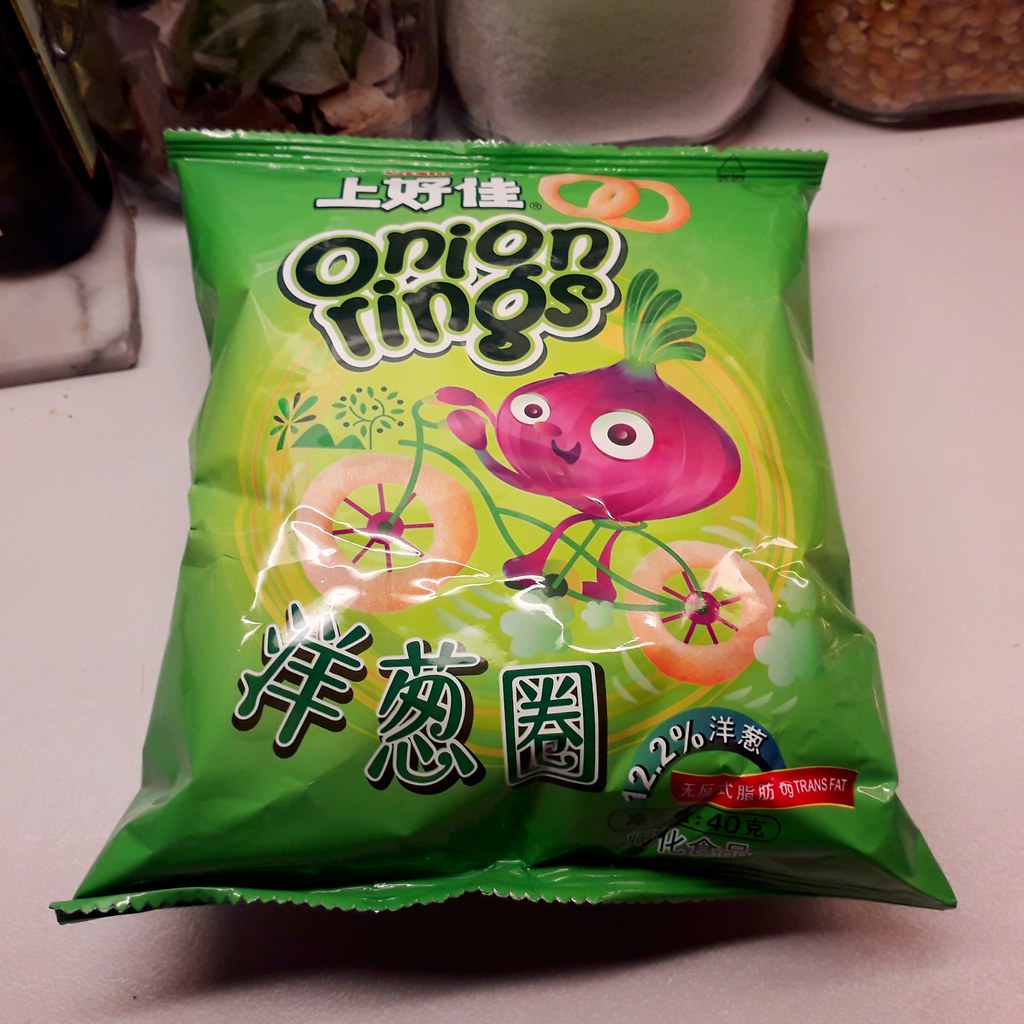This image features a vibrant green bag of Chinese snack chips labeled "Onion Rings" in large black font bordered in white. The bag lies flat on a white kitchen counter, slightly angled from the front and overhead, with its opening towards the top of the image. Surrounding the top edge of the bag is white Chinese lettering. Adjacent to this, on the right, there are two detailed onion rings.

Dominating the center of the bag, the background shifts to a bright yellow, highlighting a whimsical illustration of a pink onion with anthropomorphic features—complete with pink arms and legs, green leafy "hair," and a cheerful face. The onion character is depicted riding a green bicycle with onion rings as wheels that have purple spokes, creating a dynamic feel with small trails of smoke emanating from the tires.

In the left section of the image, more Chinese text is visible just below the bicycle illustration. The bottom right corner of the bag features a blue arch design with the number "12.2%" written in both Chinese and English, above a red banner with additional Chinese script.

The background subtly includes parts of glass jars, possibly containing dry goods, adding to the domestic kitchen setting. The scene's composition effectively centers on the colorful and playful snack packaging, merging cultural text and imaginative artwork.